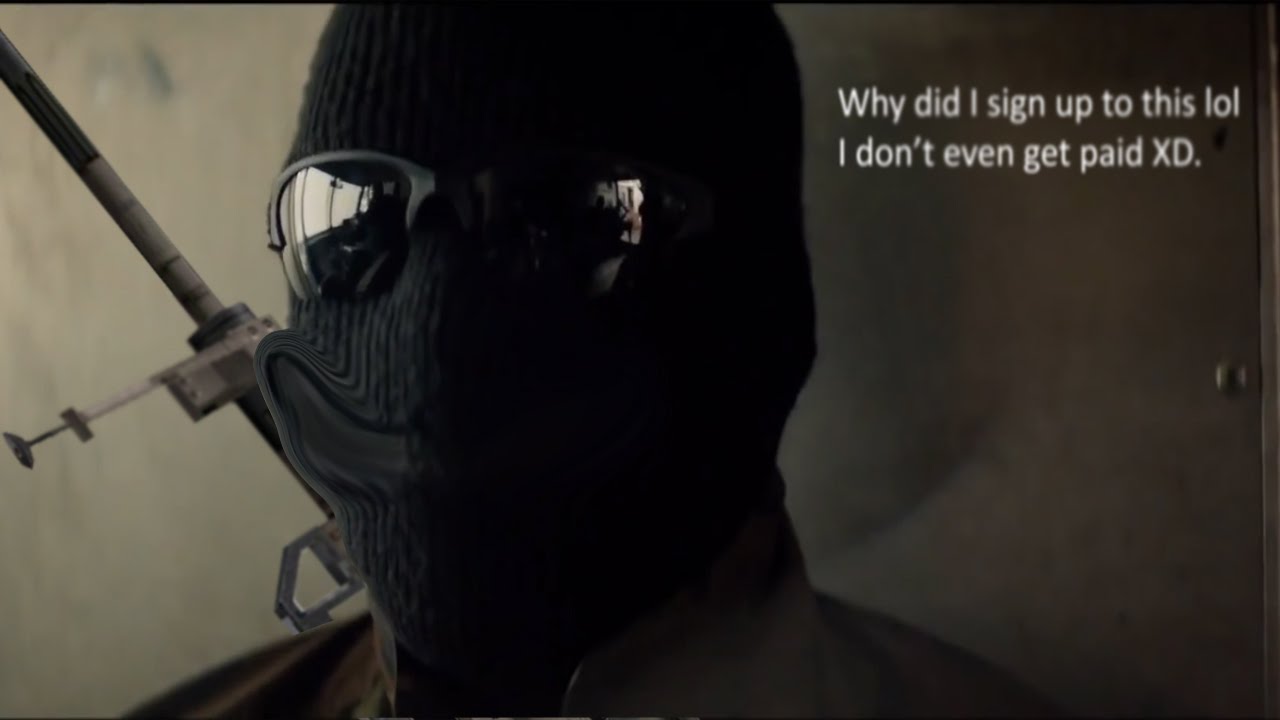In this horizontally rectangular image, the background transitions from a darker gray on the right to a lighter brownish tan on the left, providing a gradient backdrop. The focal point of the image is a head covered entirely by a knitted ski cap, obscuring the individual's facial features. Atop the ski cap, they are wearing mirrored sunglasses with black frames, reflecting the ambient light. Angling upwards towards the top left corner of the frame, the barrel of a rifle is visibly emerging from behind the individual, suggesting a sense of readiness or alertness. Overlaying the upper right portion of the image in white text are the words: "why did I sign up to this lol I don't even get paid XD," where "XD" represents a laughing face emoticon from an era before emojis. The combination of elements in the image raises questions about the circumstances and emotions experienced by the subject.